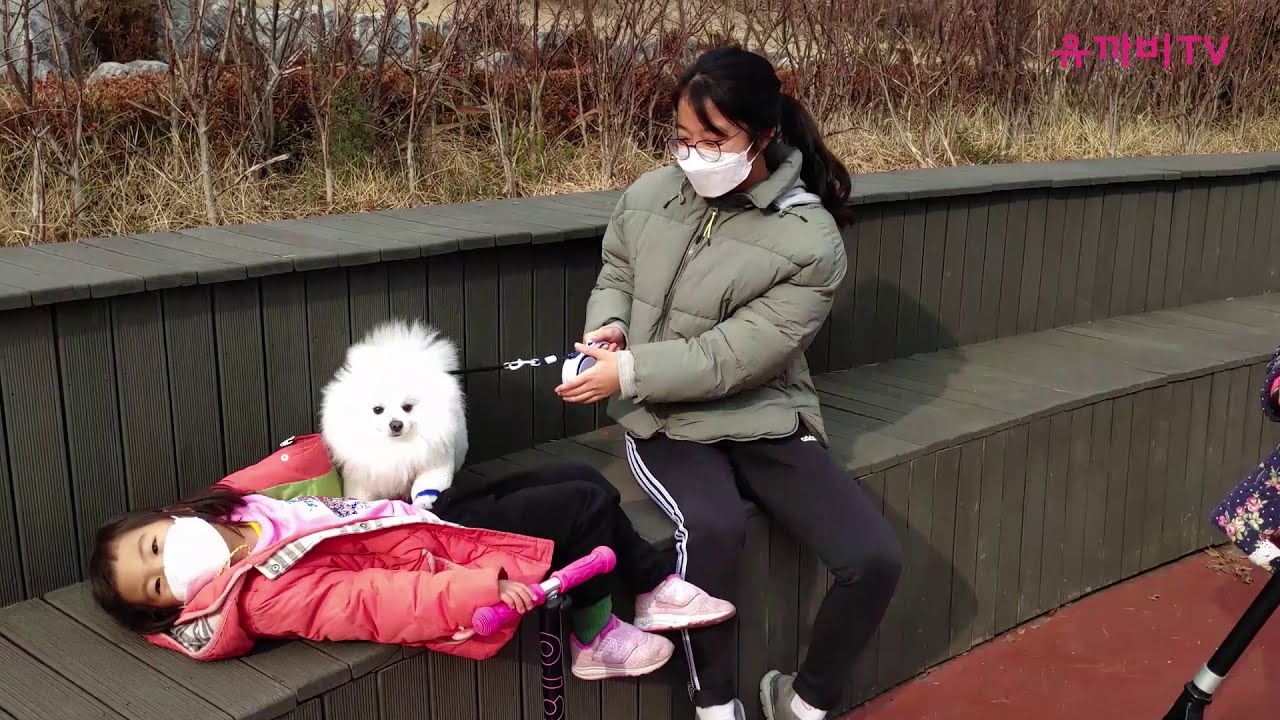The image depicts a serene outdoor scene, likely at a park on a sunny day. The setting includes a clay or stone floor that covers the bottom-right corner of the frame. At the center of the image, a woman sits on a bench that spans the entire width of the photo. She dons a gray bubble jacket, black Adidas pants, and tennis shoes, her hair pulled back in a ponytail, and wears a COVID mask. Directly beside her on the left, her daughter is lying on her back atop the bench. The little girl is dressed in a pink coat, a white COVID mask, a white and pink shirt, black pants, and white tennis shoes. She appears to be playing with a white Pomeranian dog, which is standing on its hind legs with its front paws on the child's stomach. The dog is held in place by a retractable leash grasped tightly in the woman's right hand, and additionally steadied by her left leg.

Flanking the bench are patches of greenery with grass and some bushes observable in the distance. Some text, written in an unfamiliar language, is visible in the upper right corner of the image. The overall scene is vibrant with splashes of colors such as red, black, silver, gray, purple, pink, white, green, brown, and yellow, enriching the vibrant midday ambiance and suggesting a cheerful interaction among the family members.